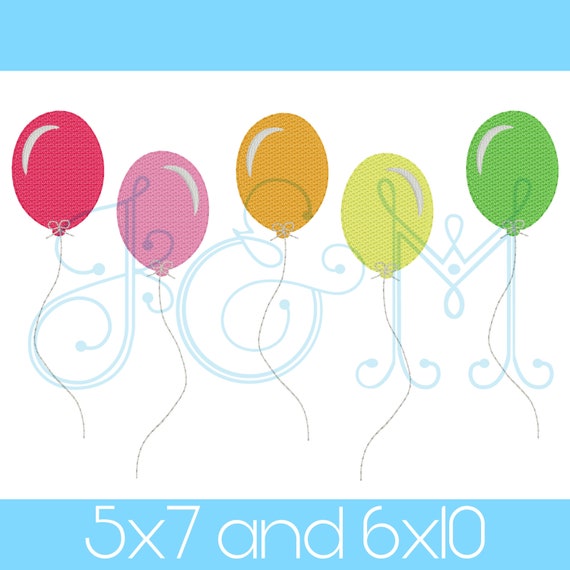The image is a square graphic with a design of five animated balloons in the center against a white background. Each balloon has a slight texture, resembling embroidery. They are arranged in a staggered vertical row with wavy blue strings hanging from each. The balloons are colored red, pink, orange, light green, and a slightly darker green. The graphic is framed with light blue bars at the top and bottom, each occupying about 10% of the graphic's height and spanning its width. The top bar is empty, while the bottom bar features centered white text reading "5x7" and "6x10" in very thin letters. Additionally, there is a decorative watermark in the middle that appears to read "J & M" in curly, light blue text.